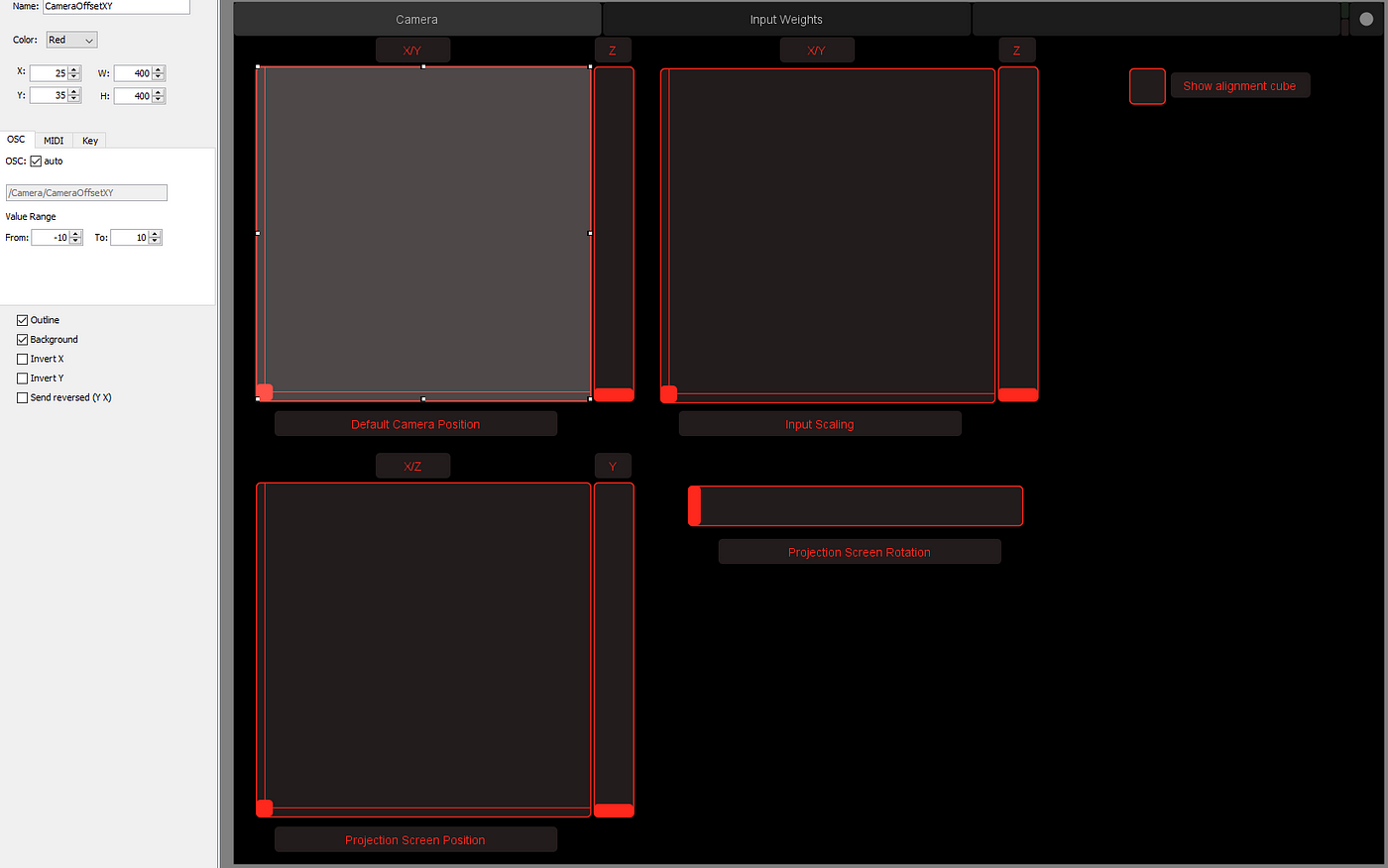The image displays a computer screen featuring an application interface. The background of the screen is predominantly black. In the center, there are three separate boxes outlined in red; the top box is rectangular, transitioning from light gray to darker gray inside. Below each box, there is red text, though it is illegible due to the image's blurriness.

On the side of the screen, a vertical menu can be seen, though its contents are unclear. There appears to be a checkbox next to one of the boxes, again accented in red. Due to the blurriness and lack of clear identifying marks, the purpose of the application remains undefined. The overall effect gives the impression of a user interface within a program rather than a website, with no clear indications or labels visible to provide further context.